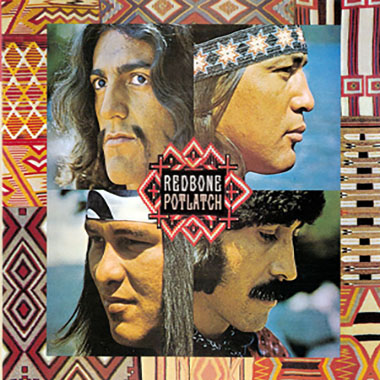This is a full-color album cover for Redbone's album "Potlatch," characterized by its vivid Native American artistic beadwork designs framing the image. The square cover is divided into four quadrants, each featuring a photograph of one of the band's Native American members. 

In the top left quadrant, a man with a Fu Manchu-style mustache gazes off-camera. Opposite him, in the top right, is a man adorned with a blue bandana decorated with white stars. The bottom left features a man with long hair tied back by a white bandana with blue stripes, and the bottom right showcases an individual with a thick, full mustache and long, wavy brown hair. The intricate border around the photographs includes red, yellow, brown, gray, burgundy, and white patterns, featuring diamonds and other motifs reminiscent of Native American blankets or tapestries, providing a rich visual context that complements the band's heritage and artistic expression.

In the center of the cover is the band's logo, "Redbone," with the album title "Potlatch" prominently displayed. This design is accentuated by red diamonds outlined in white, with the intricate beadwork underscoring the band's cultural roots. The overall composition melds together traditional Native American art with the band's vibrant musical identity.